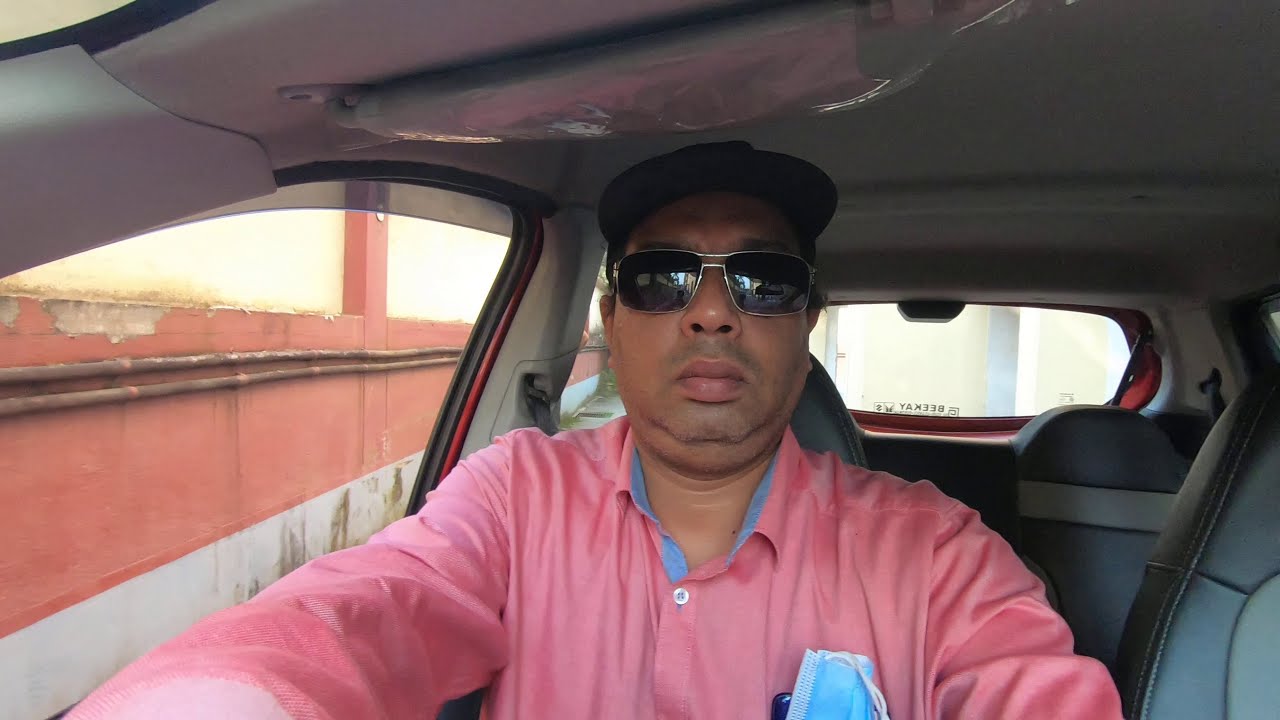In this photo, a man with a tan complexion, potentially Hispanic, sits in a car, possibly an SUV or van. His expression is neutral, with no visible smile. He has a double chin and sports facial hair, including mustache growth on his lips and chin. The man is wearing dark sunglasses and a black baseball cap. His outfit consists of a long-sleeved, pink or salmon-colored button-down shirt with aqua blue accents around the collar. A blue medical mask is tucked into his shirt pocket. The car's interior is a mix of gray, white, and black, and the seat belt is visible. The vehicle is parked next to a building that has a distinctive pink color with white structural elements and electrical conduit on its side. Additionally, the building features a red horizontal stripe with attached wires. Through the back windshield of the car, some writing is visible on a sticker.